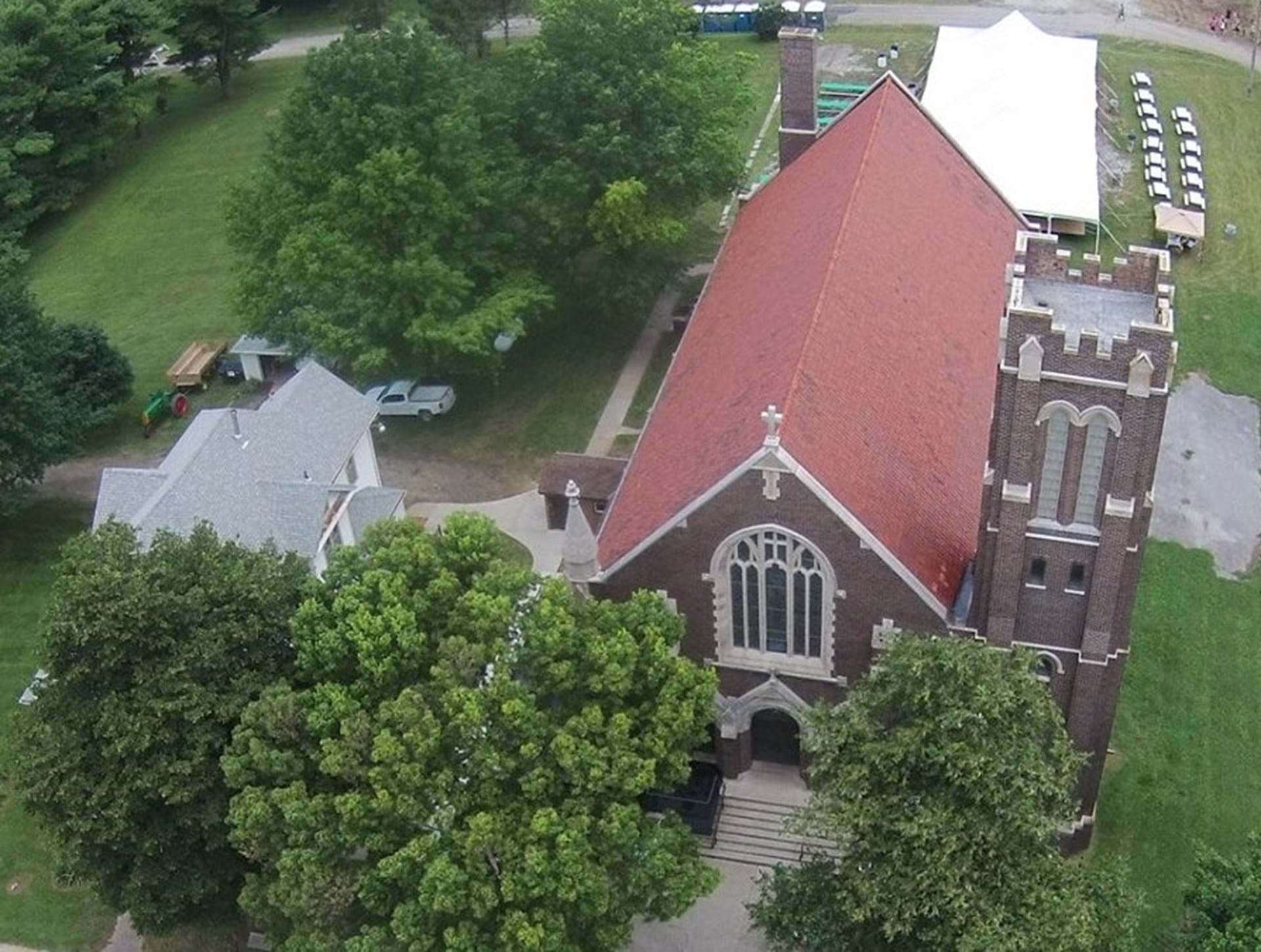This aerial photograph captures a small brick church with a red roof situated in a scenic countryside setting. The church features a prominent large arched window above its main entrance and a staircase leading down to a tree-lined cement walkway. There's a distinctive cross at the peak of the roof. To the right of the building stands a tall bell tower that rises above the church's peak, culminating in a turret area. Surrounding the church are various elements that add to its rustic charm. Adjacent to the church on the left side is a house, likely the minister's residence, with a small parking area containing several pickup trucks and a white truck in front of a garage. There's also a tractor hooked up to a trailer nearby. In the background, a low white structure, possibly used for events, includes a tent and outdoor seating arranged on the lawn. The landscape is dotted with various smaller buildings, patches of grass, and is framed by abundant trees, adding a quaint and tranquil atmosphere to the scene.